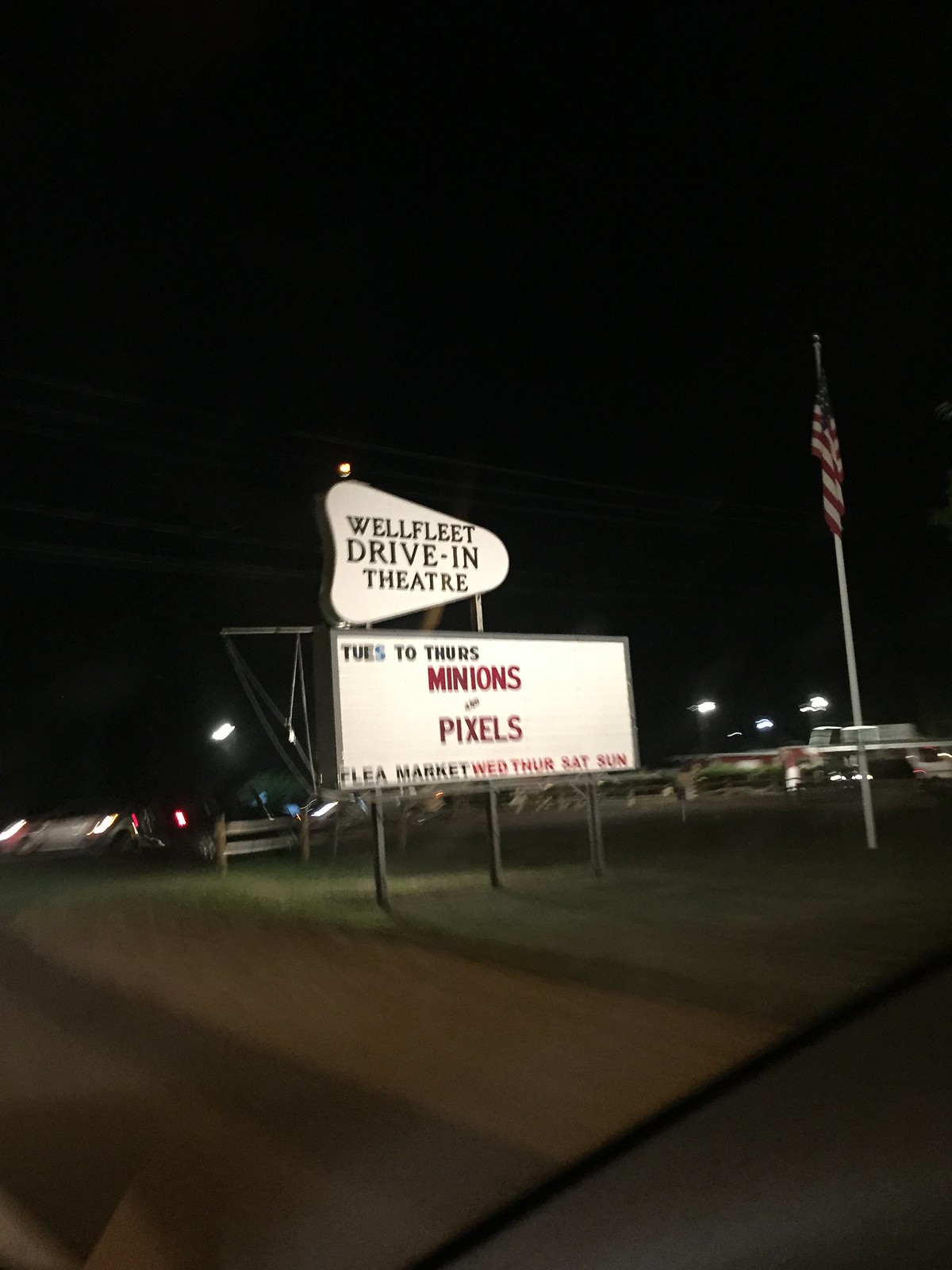The image features a billboard and sign for the Wellfleet Drive-In Theater. The sign is predominantly white with black numbers, designed in a shape reminiscent of a softened arrowhead, similar to the Sonic logo. Above the billboard, the theater announces its upcoming movie showings: "Minions" and "Pixels," scheduled from Tuesday through Thursday. Additionally, the sign advertises a flea market taking place on Wednesday, Thursday, Saturday, and Sunday. 

The sign itself is approximately five feet tall. The scene is set at night, illuminated by various lights, with cars visible in the background. An American flag on a white flagpole is prominently displayed, adding a patriotic touch. The drive-in is accessed via a dirt road, with a hint of pavement visible in the corner. Despite the rarity of drive-in theaters today, this modern venue showcases relatively recent films. However, the screen itself is not visible in the image.